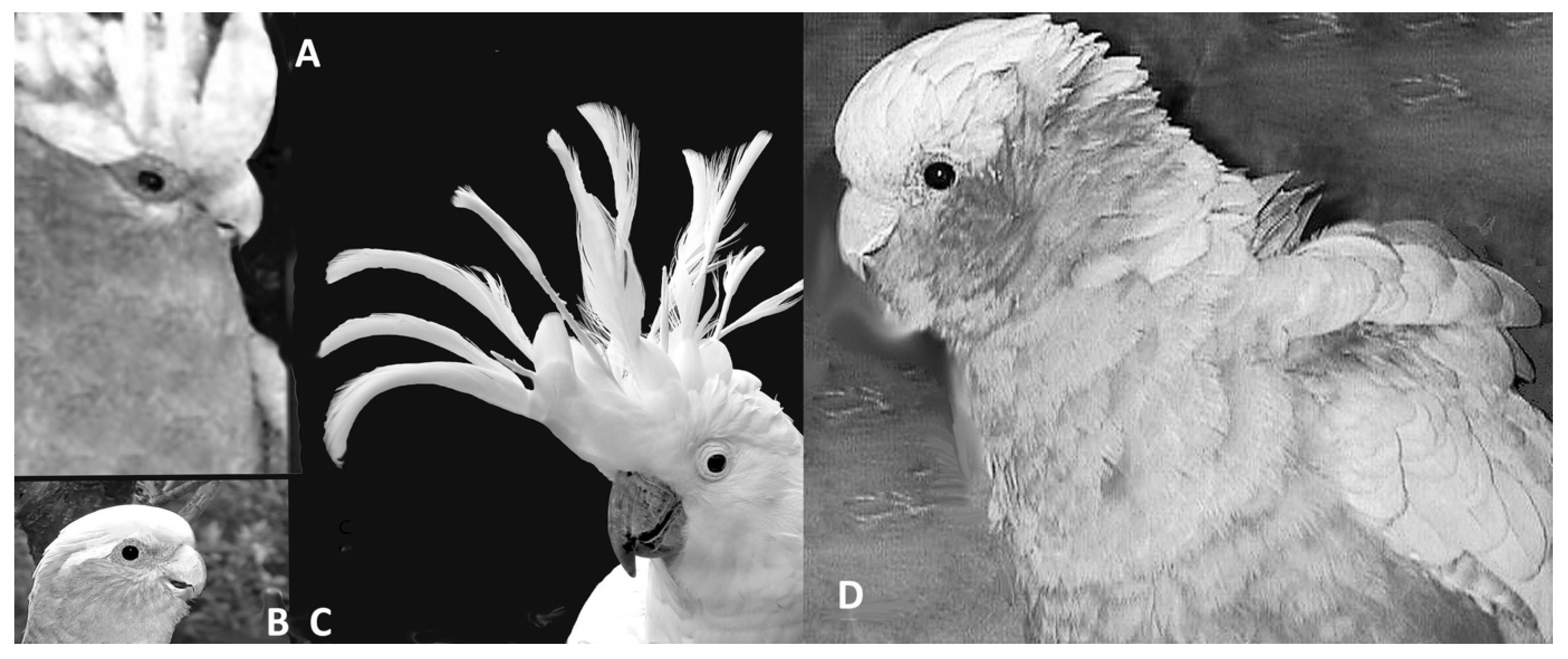This black and white collage features four distinct birds, each labeled A, B, C, and D. Image A captures a somewhat grainy profile shot of a bird with a prominent mohawk of feathers adorning its head, similar to a cockatiel's crest. Below it, image B shows a similar bird, but without a crest, presenting a more subdued appearance with a short beak and a midway gaze. Image C stands out with a white bird set against a black background, displaying a comical expression and a dramatic flourish of feathers on its head that resembles a major mohawk. Finally, image D depicts a smaller bird with a more relaxed and tidy appearance, giving a side profile view with no protruding feathers. The images, though varying in quality and clarity, collectively showcase the unique characteristics and personalities of each bird.